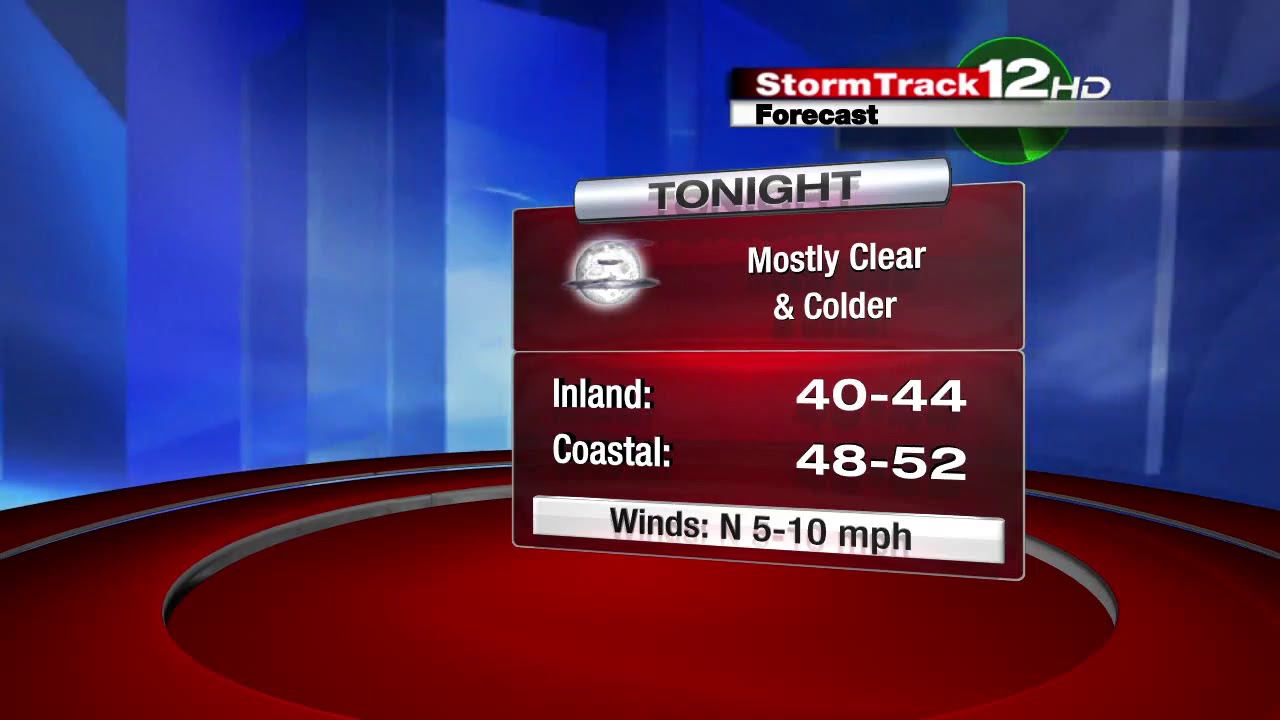The image appears to be a frame from a news program capturing a detailed weather forecast graphic. The background features abstract blue 3D shapes that resemble buildings. On the upper right, there is a green circle with the "12 HD" logo and a "Storm Track Forecast" label. Below this, a layered red and silver panel displays the forecast for tonight. The silver box includes an icon of a moon on the left side, next to the text "mostly clear and colder." Information about temperatures is divided into two sections: "Inland" with a range of 40 to 44 degrees Fahrenheit, and "Coastal" with a range of 48 to 52 degrees Fahrenheit. Beneath this, a smaller white box provides details about the winds, indicating speeds from 5 to 13 miles per hour.